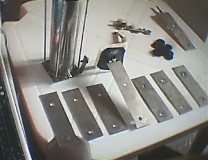In this detailed image, we see a small, indoor scene centered on a white surface that could be either a table or a workbench, possibly made of thick plastic. Across the front edge of the workbench lies a series of six metallic silver rectangles, each with a single hole punched at both ends. These rectangles are oriented perpendicular to the edge of the table. The middle rectangle is slightly different: it's a lighter color, appears longer, and is raised at an angle.

In the background, there's a tall, cylindrical object, shiny and smooth, possibly made of silver or gray material. This cylinder stands upright and extends off the edge of the picture, and there are thinner poles running parallel to it, though not touching it. Scattered around the table are small tools and accessories that suggest they could be used to install the metal bars onto something. The overall image provides a sense of a work area with various components neatly arranged, indicating ongoing or potential assembly work.